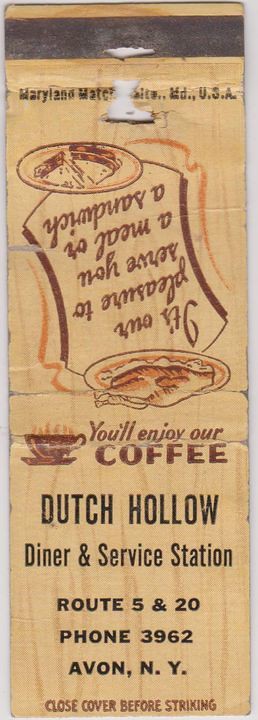The image depicts a vintage matchbook advertisement from the Dutch Hollow Diner and Service Station located at Route 5 and 20, Avon, New York, with a phone number, 3962. The matchbook is worn, showing signs of age with dog-eared edges, scratches, and bending. The design includes a prominent slogan, "You'll Enjoy Our Coffee," accompanied by an illustration of a steaming coffee cup. Due to the matchbook being laid flat, the top half appears upside down. This section features a menu adorned with images of a turkey or chicken dinner on a platter and a sandwich on a plate, alongside partially obscured text stating "It's our pleasure to serve you a meal or a sandwich." Adding to the authenticity of its vintage appeal, the matchbook carries the common safety warning, "Close cover before striking," reflecting its probable era from the 1950s or 1960s.